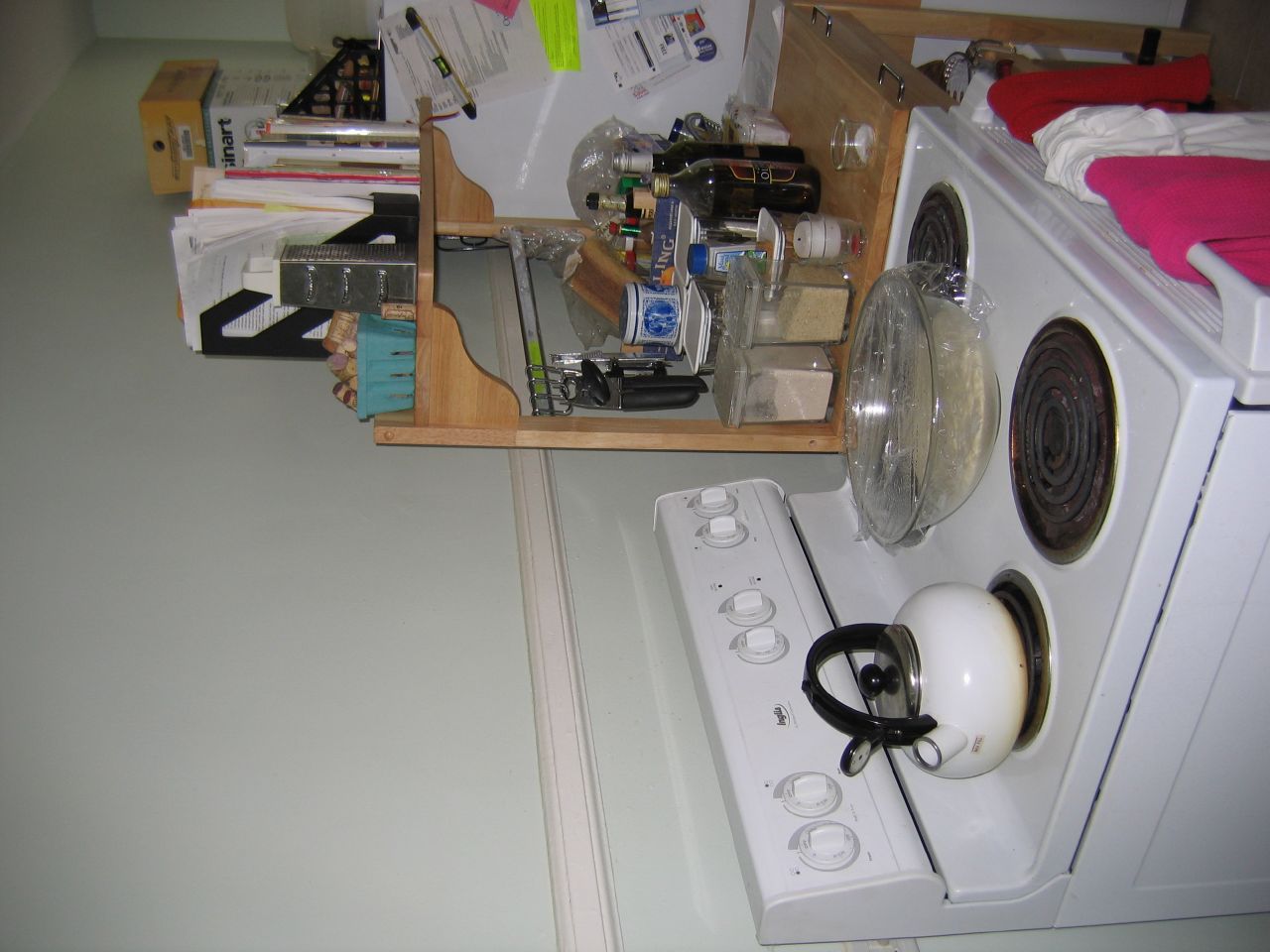This photograph captures a cozy kitchen corner in vivid detail. The upper left corner of the image features a plain white wall adorned with a simple white molding strip across the middle. Dominating the lower left portion is a pristine white stove, equipped with four black burners. On the upper left burner, a white tea kettle with a black handle rests, ready for use. Centrally positioned on the stovetop is a large, translucent glass serving dish, its beige contents sealed under a layer of plastic wrap.

Adjacent to the stove is a light wood rack brimming with kitchen essentials. The rack holds an array of spices and several bottles of olive oil. Two large canisters, one filled with white powder and the other with beige powder, stand prominently. A small white tea light candle adds a touch of warmth to the scene. The shelf also contains a collection of papers, neatly organized in little black cases.

In the backdrop, a white refrigerator features a collage of papers and notes, adding a personal touch to the kitchen space. Adding a splash of color, three towels in pink, white, and red hang from the oven door handle, ready to assist with any culinary task.